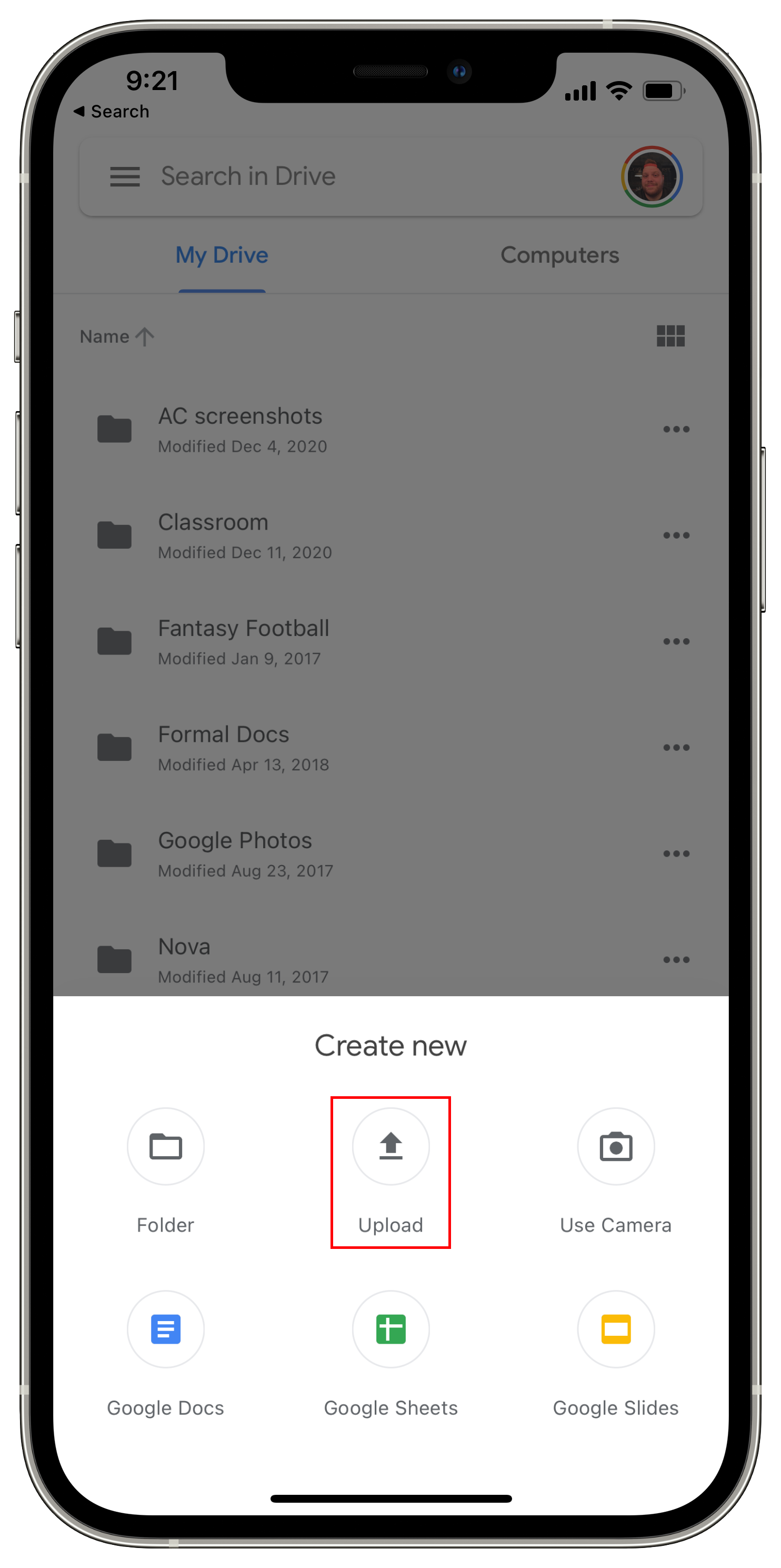The image depicts a mobile device with a sleek black trim and a silver or clear metallic exterior. The screen shows the user viewing their Google Drive, which displays a white background. At the top of the screen, there is a prominent search bar, identifiable by its rectangular shape and the text "search in Drive" written in gray with three gray lines on the left. On the right side of the search bar, there's a user icon featuring a male avatar, likely with red hair, surrounded by the Google color border.

Directly beneath the search bar, the text "My Drive" and "Computers" is visible, with "My Drive" highlighted in blue and underscored by a matching blue line. Below, the display lists various folders, beginning with a folder labeled "AC" in capital letters, followed by another one named "Screenshots." The "Screenshots" folder is annotated with a modification date of "DEC 4, 2020" in small gray lettering. 

This interface appears semi-transparent as it overlays a menu of new settings at the screen's bottom. At the center of this overlay, in a rounded Sans Serif font, the words "Create New" are written in gray. Several options are presented here, with the "Upload" option emphasized by a red rectangle. This specific option features a circular light gray border enclosing a thick medium gray arrow pointing upwards with a line underneath it. To the left of this is another icon, also in a circular light gray border, depicting a gray folder shape with the word "Folder" written beneath it.